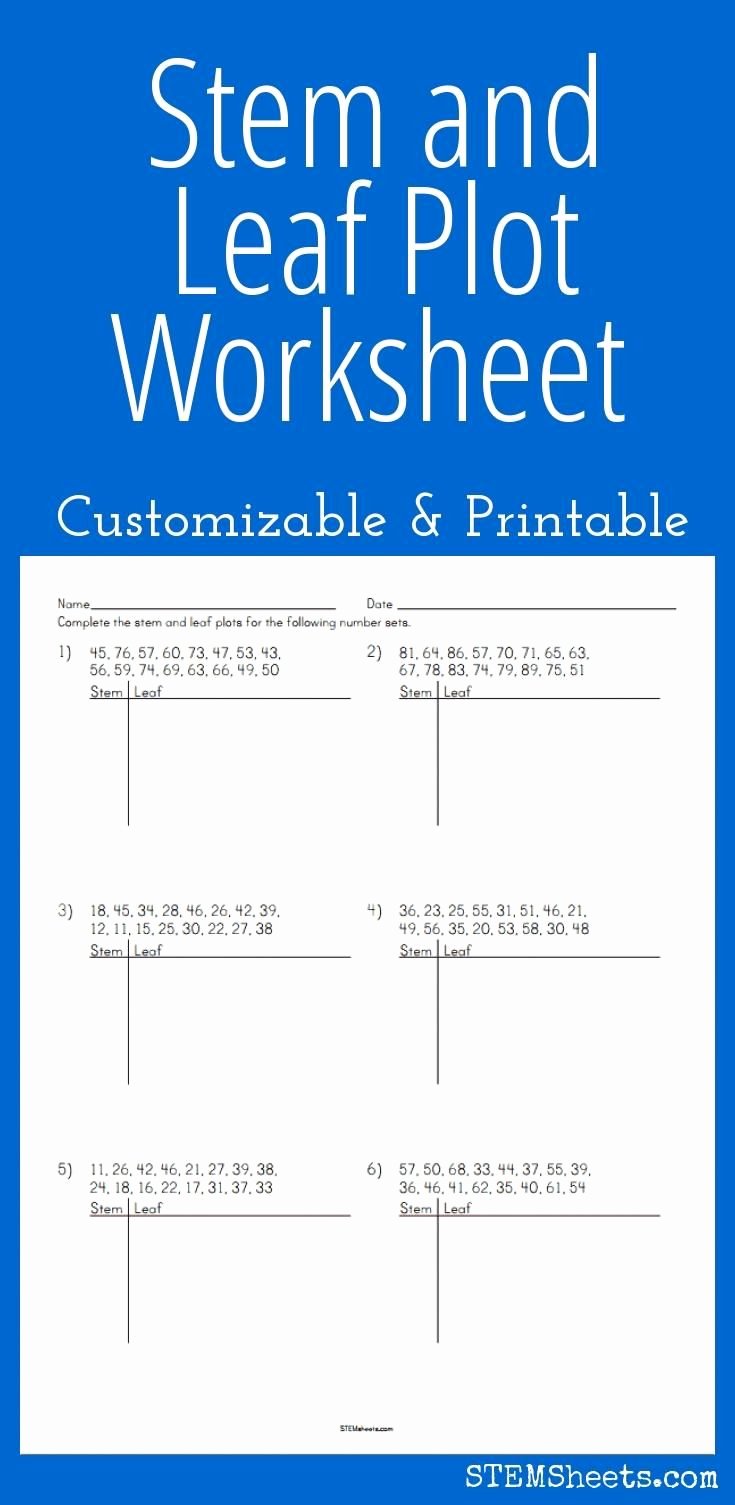This image represents a vibrant blue, vertical rectangle worksheet designed for math practice, specifically focusing on stem and leaf plots. At the top, in clear white letters, it reads "Stem and Leaf Plot Worksheet - Customizable and Printable." Directly below this header, there is a white rectangular space designated for user input, with fields labeled "Name" and "Date," followed by six enumerated problems. Each problem contains a sequence of numbers, separated by commas, intended for the creation of stem and leaf plots.

The worksheet instructs students to complete these plots, with columns titled "Stem" and "Leaf," demarcated by a vertical line and underscored by a horizontal line for clarity. Problems are balanced across the sheet, with three on the left and three on the right. Finally, in the bottom right-hand corner, the source "stemsheets.com" is discreetly printed in small white text, emphasizing the worksheet's availability for printing and customization.